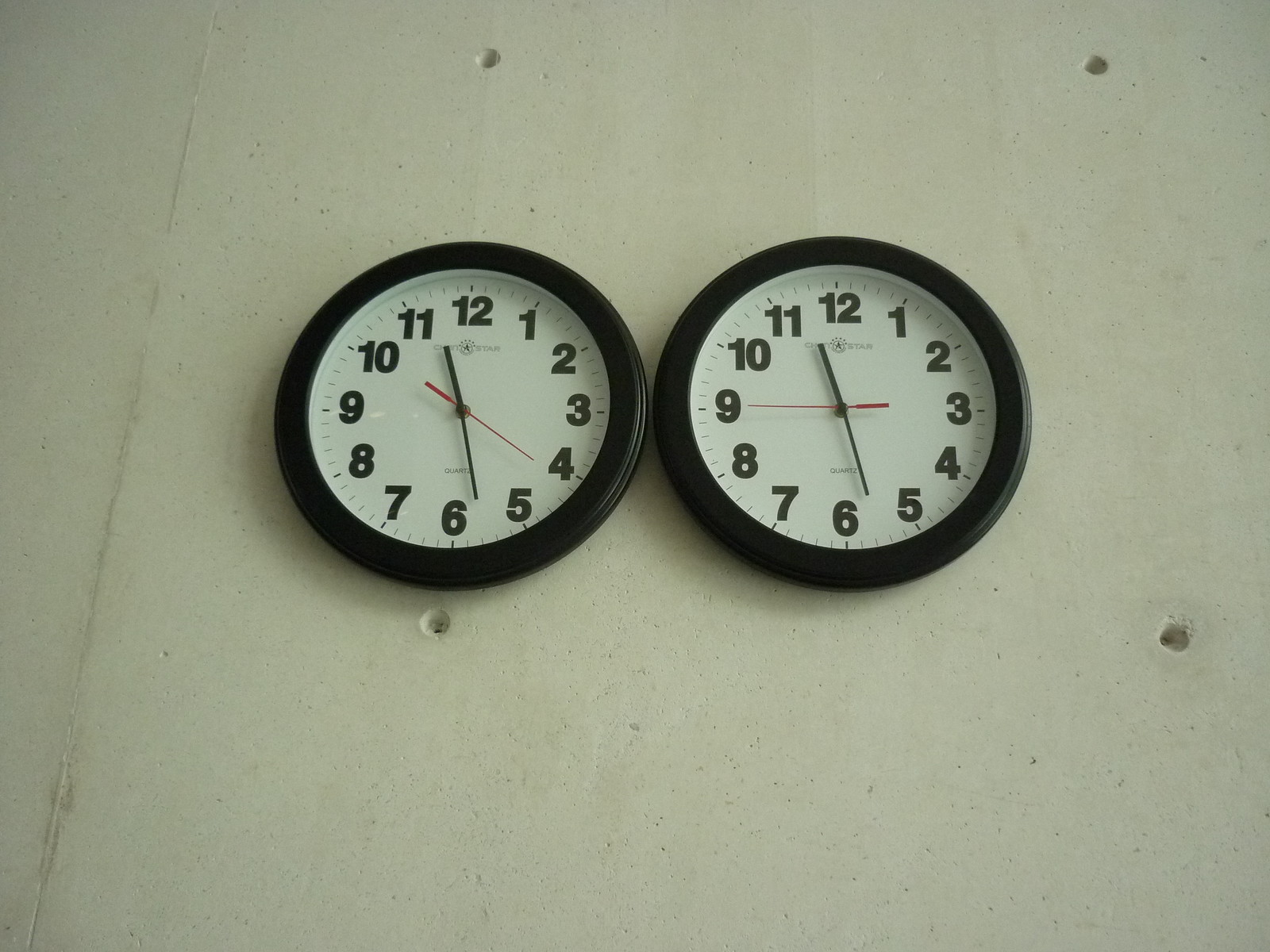A pair of identical wall clocks, both reading 11:29, is prominently displayed in the image. Each clock features a black border, with black numerals marking the hours and black hands signaling the minutes and hours, complemented by a red second hand. The clocks appear to be mounted on a wooden wall, aligned closely together, almost touching. The angle of the photo, taken from above, gives a clear view of the clocks' faces and emphasizes their synchronized time. The brand of the clocks remains indiscernible in the image.